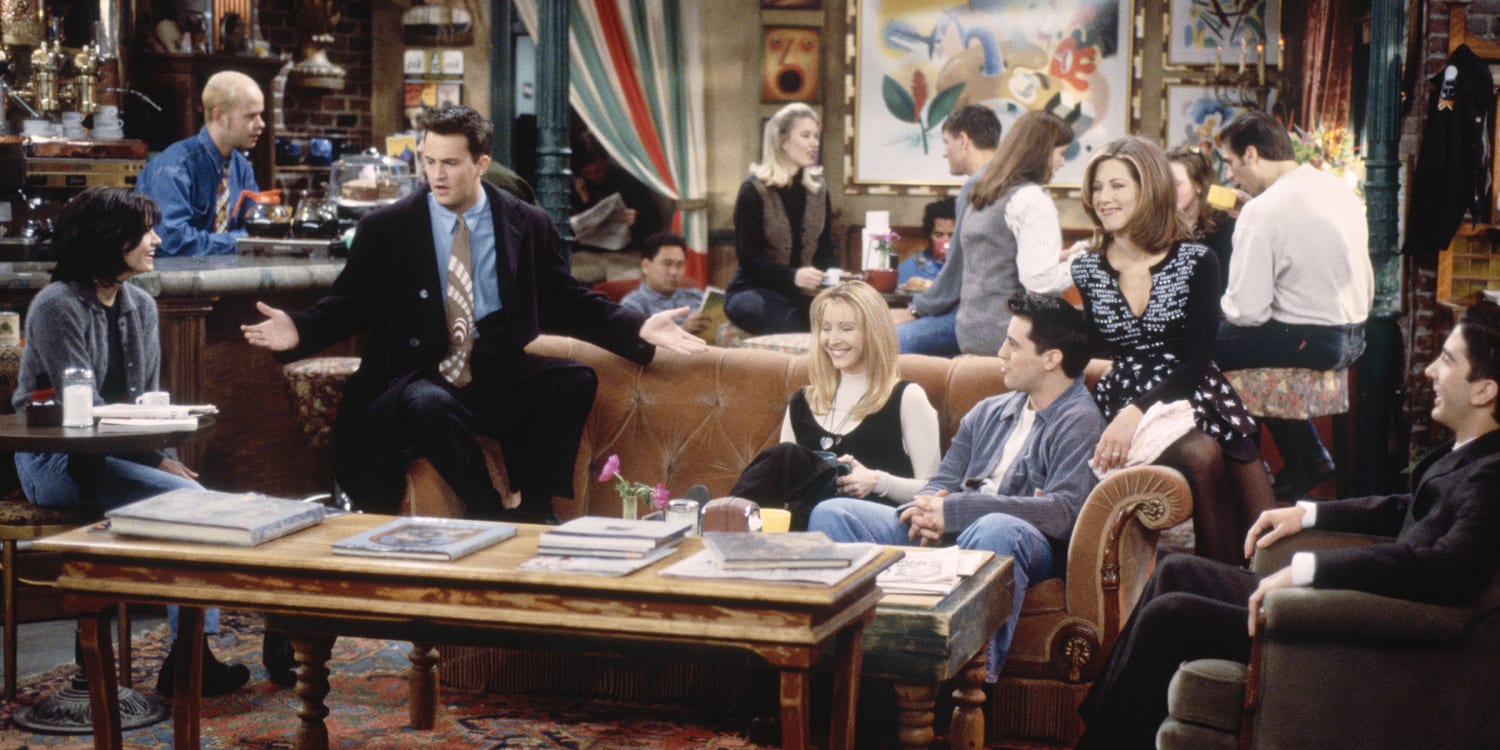The image depicts a scene from an early episode of the TV show "Friends," specifically set in the iconic Central Perk café. The main cast—Monica (Courteney Cox), Chandler (Matthew Perry), Phoebe (Lisa Kudrow), Rachel (Jennifer Aniston), Joey (Matt LeBlanc), and Ross (David Schwimmer)—are all present, indicating it's most likely from the first three seasons based on the low-quality resolution. The friends are seated on the familiar brown leather sofa, with Chandler raising his hands in a humorous gesture that captures everyone's attention. Joey and Monica are attentively looking at Chandler. The scene is lively, with happy, engaged conversations among the characters, who are joined by several crowd extras in the background. 

In the café's backdrop, a bartender can be seen behind the brown bar with a gray marble top. Central Perk’s distinctive décor is visible, including the intricate painting on the wall and the oriental rug on the floor. The café tables are adorned with details such as a white candle, books, coffee cups, and papers. Each character’s attire reflects the early '90s fashion: Chandler in a blue shirt with a beige and white tie paired with a black suit, Phoebe in a white top and brown jumper-like dress, Joey in blue jeans and a gray sweater, Rachel with her shoulder-length hair and a black and white top, and Ross in a black suit. Their outfits contribute to the colorful ambiance of the café, enhancing the overall aesthetic of the scene.